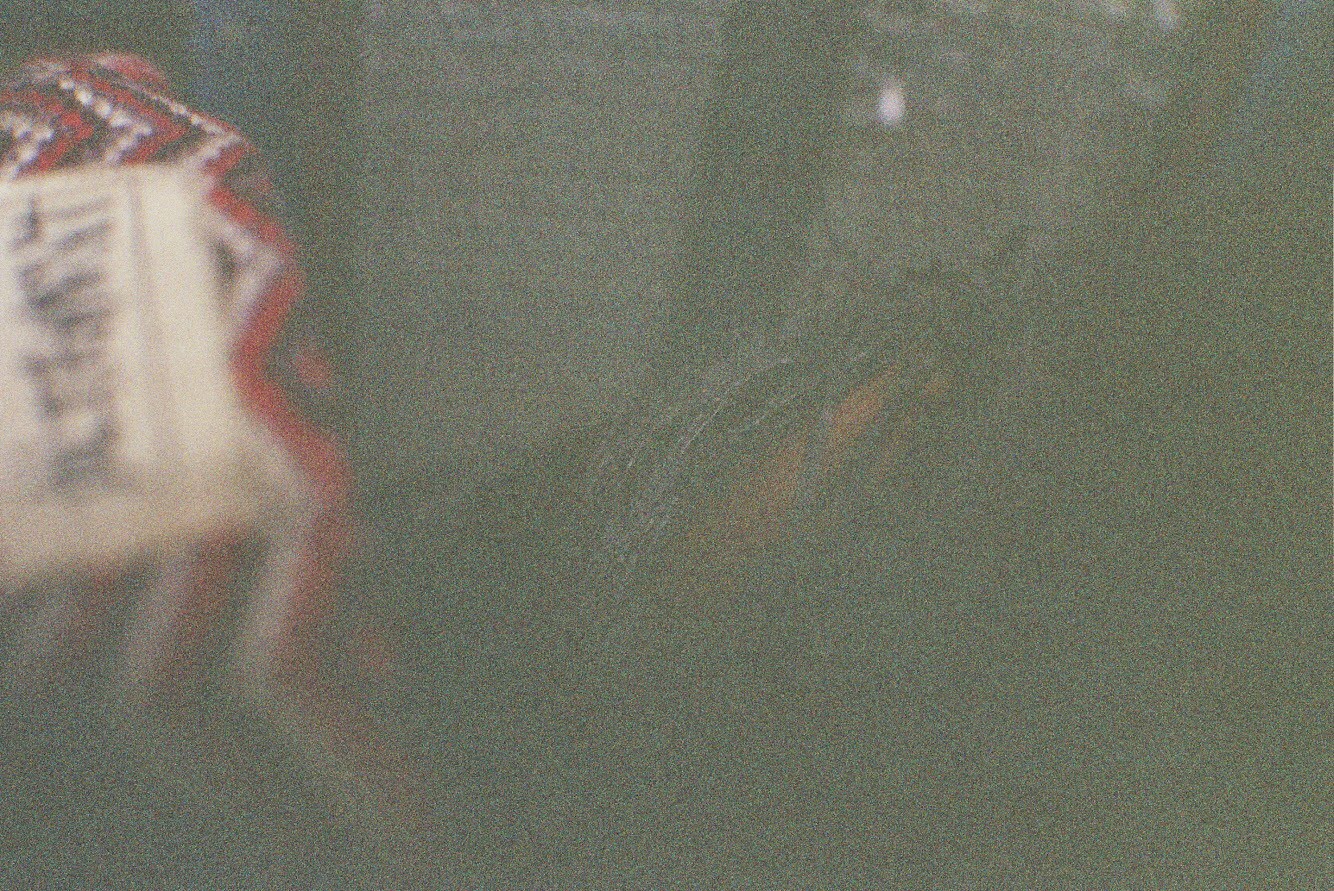A dimly-lit photograph showcasing a detailed scene on the left-hand side featuring a blanket adorned with a striking chevron pattern. The blanket exhibits alternating stripes in red, white, and black, with the pattern creating a dynamic series of upward and downward triangles. A white label with some indistinguishable black text is visible on the blanket, though it is partially obscured by the darkness. The lower quarter of the image is predominantly in shades of black and gray, providing a stark contrast to the colorful blanket. At the top of the image, a gray-colored doorway framed by brown wood trim is visible, adding an architectural element to the composition.